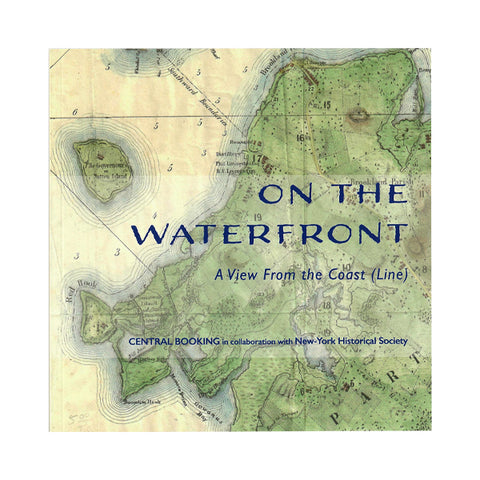The image depicts a detailed book cover featuring an old-style map illustration. Dominating the cover is a top-down view of a peninsula on the right in muted green, surrounded by waterways in blue and pale cream. To the upper left, a small island shares the same green hue. The map, densely labeled with various features, has numbers like 3, 5, and 16, although the lettering is too small to be deciphered clearly.

Overlaying the map, in bold blue font, is the title "On the Waterfront: A View from the Coast (Line)." Below the title, smaller blue letters attribute the work to "Central Booking in collaboration with the New York Historical Society." Despite the intricate details of the map, it remains challenging to determine the specific location, though it suggests a coastal landscape, possibly New York.